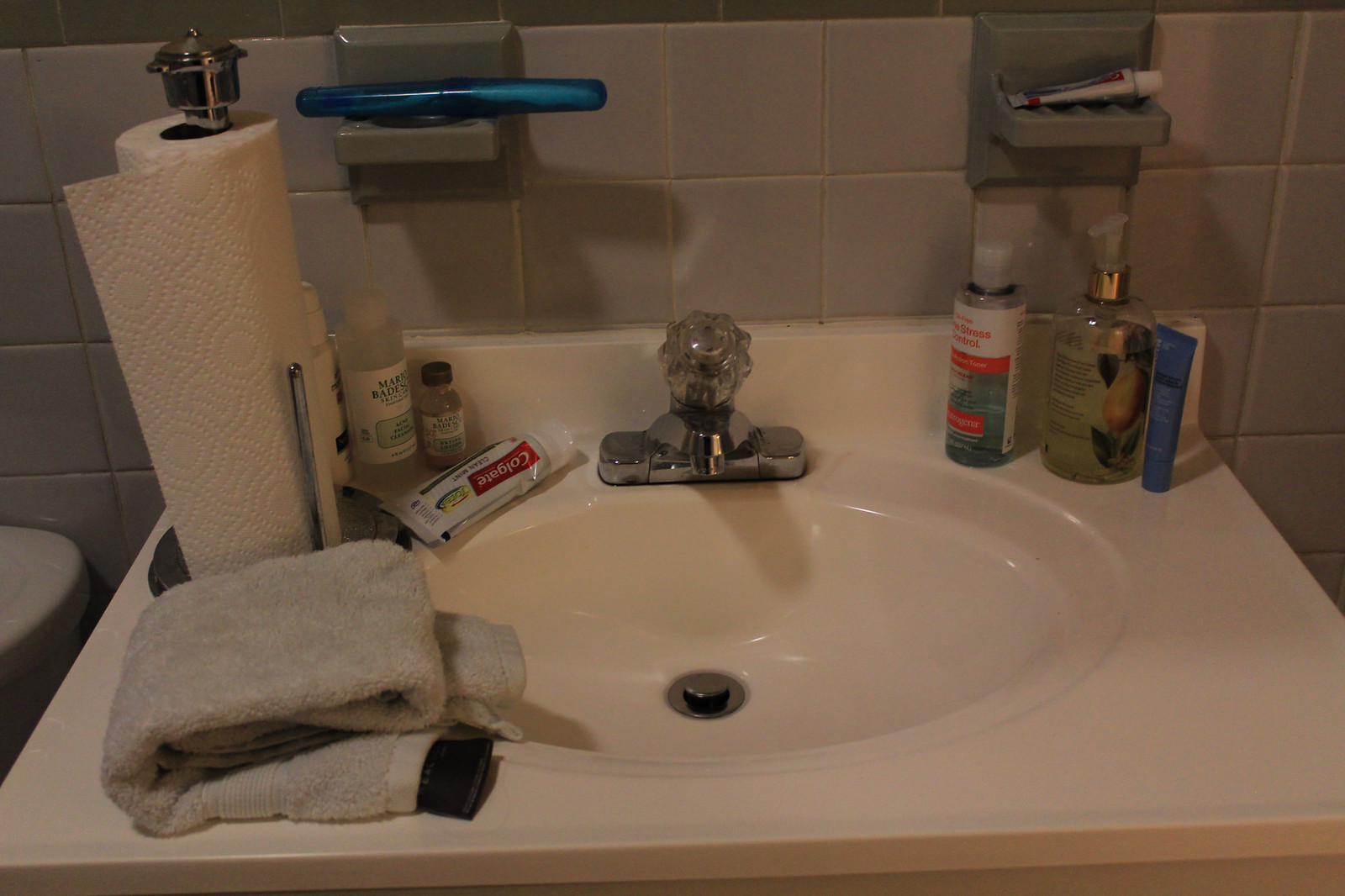This photograph showcases a somewhat dimly lit, dated bathroom sink area, characterized by a sense of aged functionality. The surrounding tiles are a light to medium gray, with visibly aged grout interspersed between them. The tiling includes two recessed sections: one designed to hold soap but currently occupied by a small tube of toothpaste, and another likely intended for a cup, featuring toothbrush holes, which presently has a blue tube of an unidentified product lying horizontally.

The sink is notably square with a circular to oval-shaped basin, suggesting a design from possibly the 1980s, though the material is uncertain. It includes a silver-tone faucet with a singular plastic knob for adjusting water temperature by turning it left or right. 

On the left side of the sink, a gray folded towel rests at the front corner. Above it is a slender, silver-tone towel rack holding paper towels upright. Further left, a tube of Colgate toothpaste is nestled between a taller plastic bottle and a smaller bottle.

On the right side of the sink, a light green hand soap pump adorned with a fruity image stands prominently, accompanied by another bottle and an additional tube. The sink basin features a silver-tone stopper, contributing to the overall dated yet utilitarian aesthetic of the bathroom space.